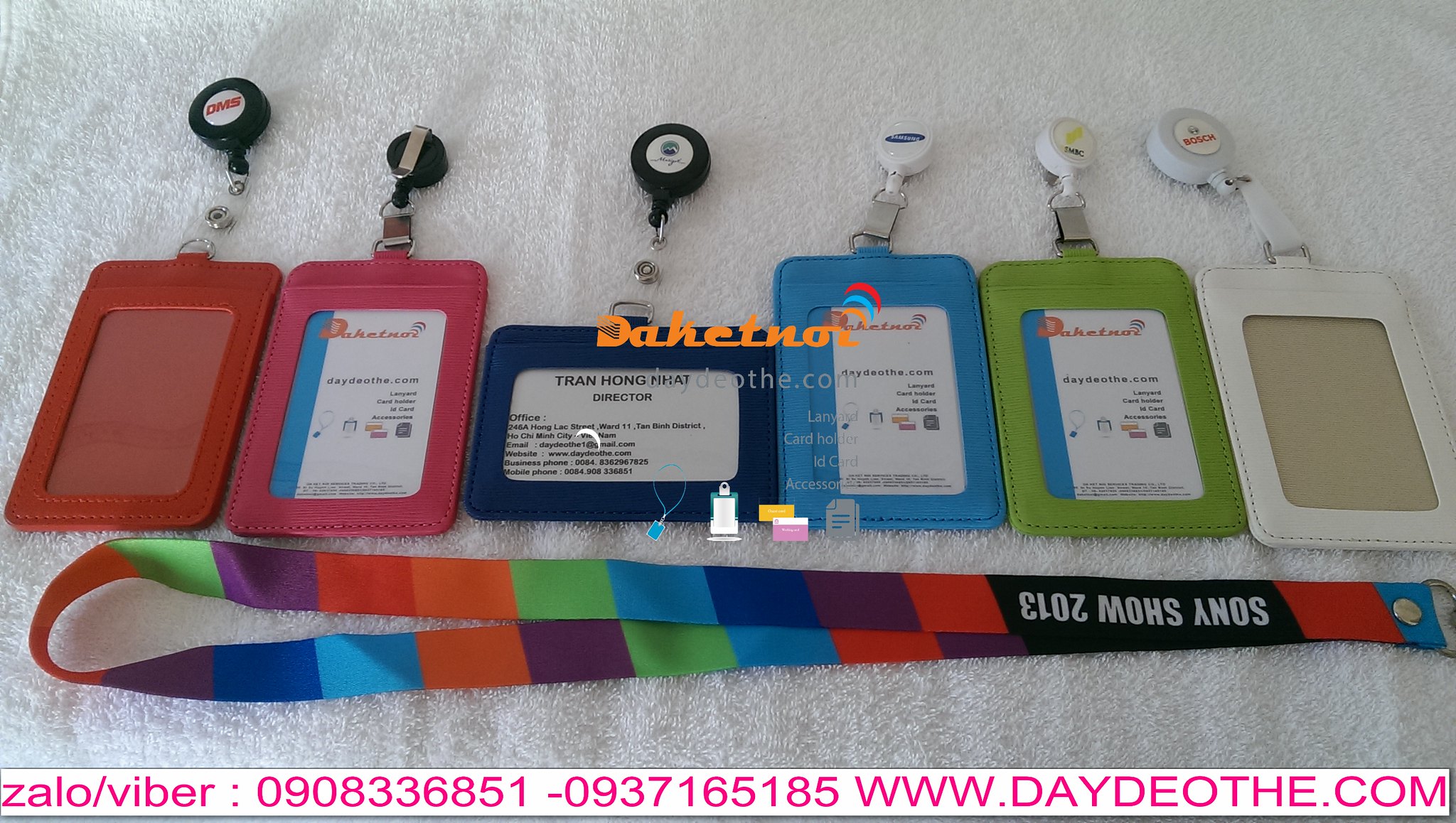The image depicts a collection of six ID lanyards arranged in a row against a white towel background. From left to right, the lanyards are in the following colors: red, pink, dark blue, light blue, green, and white. The first lanyard on the left is red with a black button on top and is empty. The second lanyard is pink, also with a black button, containing a white card with a blue border. The third lanyard is dark blue with a black button, displaying a white card that reads "Tran Hong Phat, Director." The fourth lanyard is light blue with a white button and holds a business-type card. The fifth lanyard is green with a white button, featuring a business card. The last lanyard on the right is white with a white button and is empty. Beneath all the lanyards, a long rainbow-colored tag lies horizontally, embossed with the text "Zalo/Viber: 0908-336851, 0937165185, www.daydov.com" in pink letters within a white border.